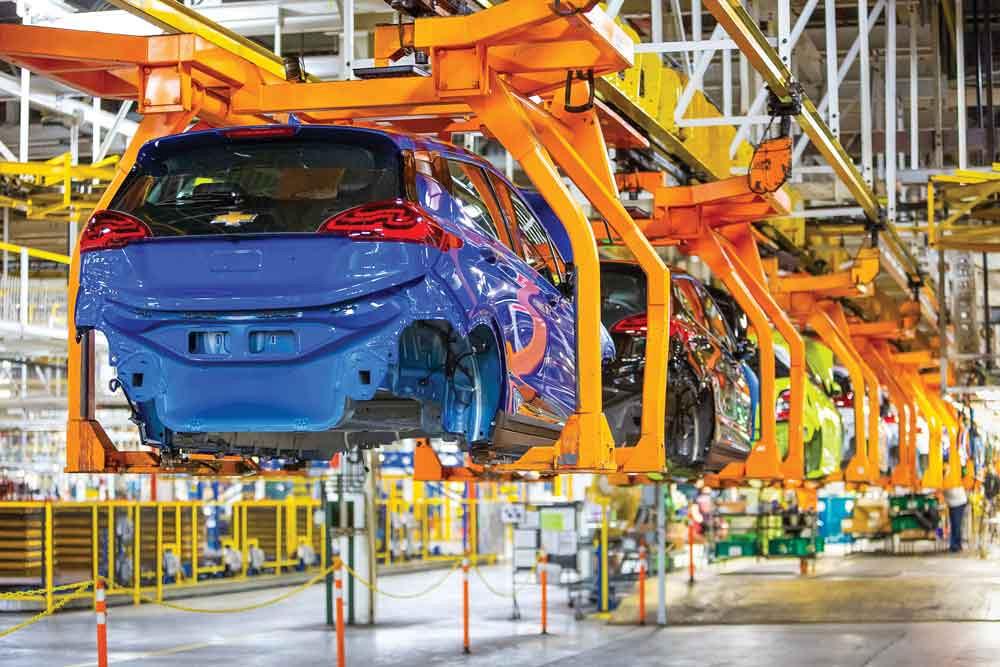This detailed image captures the interior view of a bright, expansive car factory where small economy hatchback sports cars, including blue, red, and lime green, are being assembled. In the foreground, there are two neon blue Chevrolet hatchbacks, nearly complete but missing wheels, suspended from an elevated conveyor line supported by a robust orange girder structure. The cars are held securely by yellow arms that reach down from the overhead rails. The factory is lit brightly, with beams of light illuminating the shiny, gray concrete floor. Toward the far end of the assembly line, a lone worker is visible, ensuring everything runs smoothly. The clarity and shine of the scene reflect the meticulous industrial environment of this massive automotive manufacturing plant.